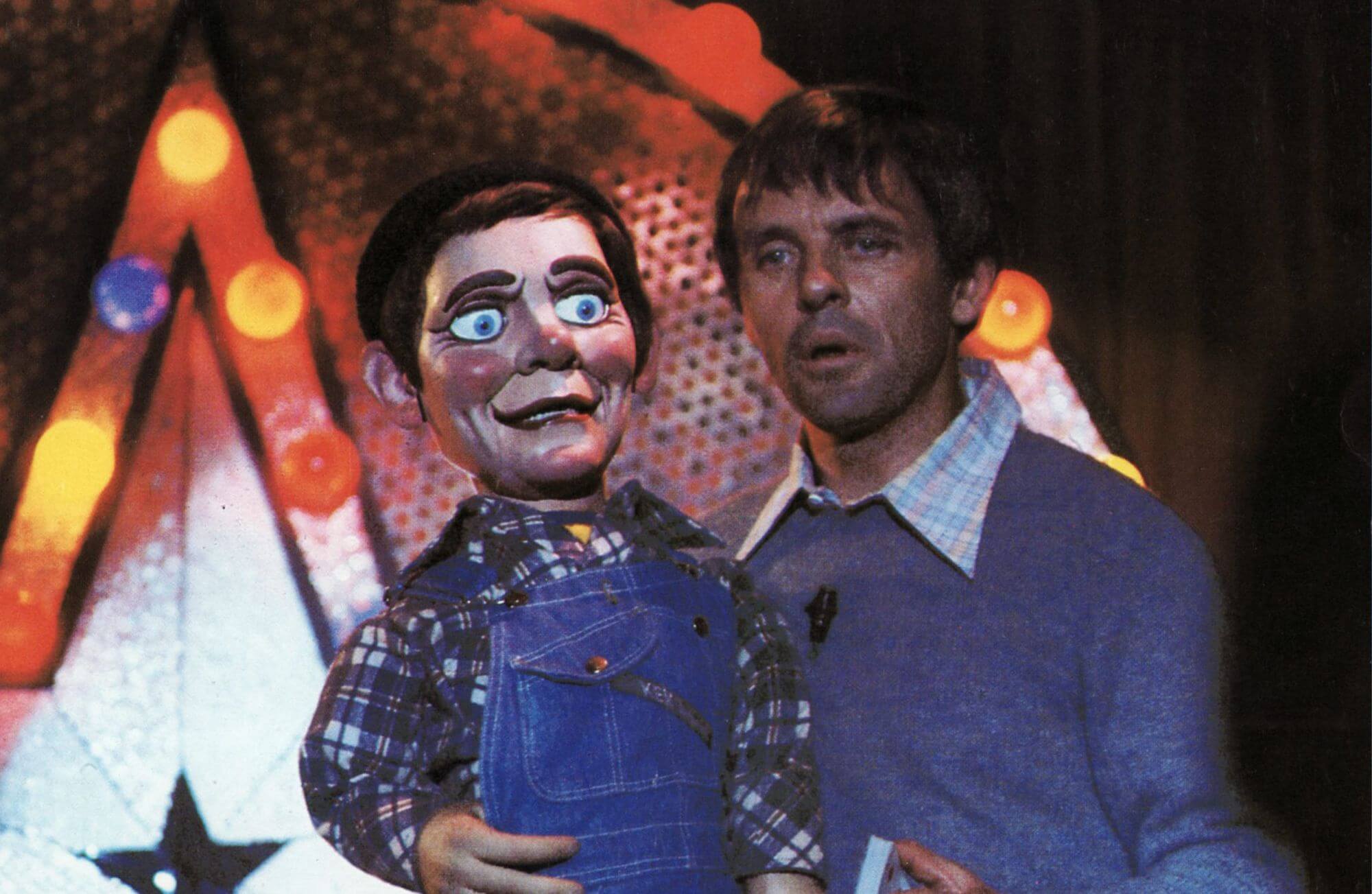In this detailed image, a young Anthony Hopkins is seen in a close-up shot, playing his role as a ventriloquist. He cradles a ventriloquist dummy on his left hand that eerily resembles him, complete with brown hair and large blue eyes. The dummy is dressed in blue dungaree overalls and a patterned shirt with shades of blue, purple, and white, matching the plaid-style attire Hopkins wears. While the dummy's shirt arrangement includes three black buttons for various purposes, Hopkins himself sports a blue long-sleeved sweater over a plaid collared shirt featuring pink, blue, and white tones. Both share the same complexion, hair color, and eye color, creating a striking resemblance between the two. Hopkins' mouth is open, depicting a surprised expression, whereas the dummy looks off to the right. In the backdrop, a large, illuminated star with a smaller black center star and multi-colored lights forms part of what appears to be a carnival or stage setting, accompanied by additional red accenting and a brown curtain. The scene is veiled in neutral, warm tones, enhancing its vintage feel, evocative of a bygone era.